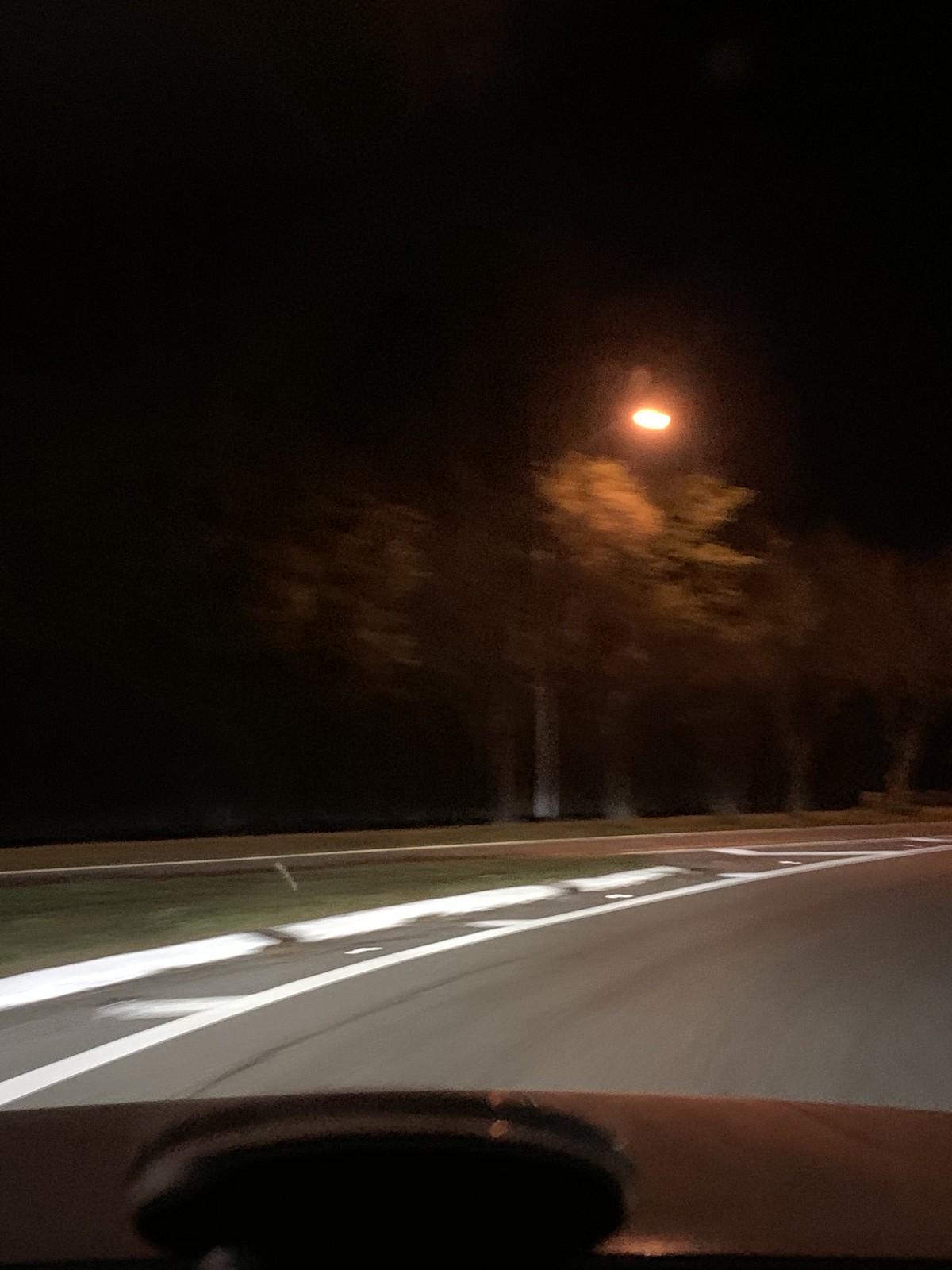Captured from the perspective of a driver, this nighttime scene reveals a dimly lit street lined with trees. The pitch-black sky serves as a backdrop to the subtle illumination provided by a solitary streetlight standing amidst the foliage. On the left side of the road, the curve of a white lane line is clearly visible as the vehicle navigates a right turn. A small grassy median lies between the lane and the intersecting road ahead. Beyond this median, a line of trees with whitish trunks and vibrant orangish-yellow leaves stands under the streetlight's glow, adding an ethereal quality to the darkened landscape.